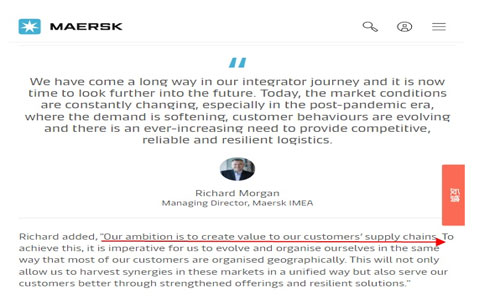This image depicts a section of the Maersk website, showcasing a well-organized and informative layout. At the top left, there is a blue icon box featuring a white star, accompanied by the text "Maersk" in bold, capitalized black font. To the right, the interface includes a magnifying glass icon for search functionality, followed by a circular icon with a drawn person indicating a profile section. Further to the right is a hamburger menu icon represented by three horizontal lines.

Beneath these elements, there is a small space followed by a body of centered text, encapsulated by quotation marks. The text reads: "We have come a long way in our integrator journey, and it is now time to look further into the future. Today, the market conditions are constantly changing, especially in the post-pandemic era where the demand is softening. Customer behaviors are evolving, and there is an ever-increasing need to provide competitive, reliable, and resilient logistics."

Below this text, there is an image of a man in a suit, identified as Richard Morgan, the Managing Director of Maersk IMEA. Adjacent to this image is an orange button with text, featuring a long right-pointing arrow that begins at the word "R" and extends until "chains" in the surrounding layout.